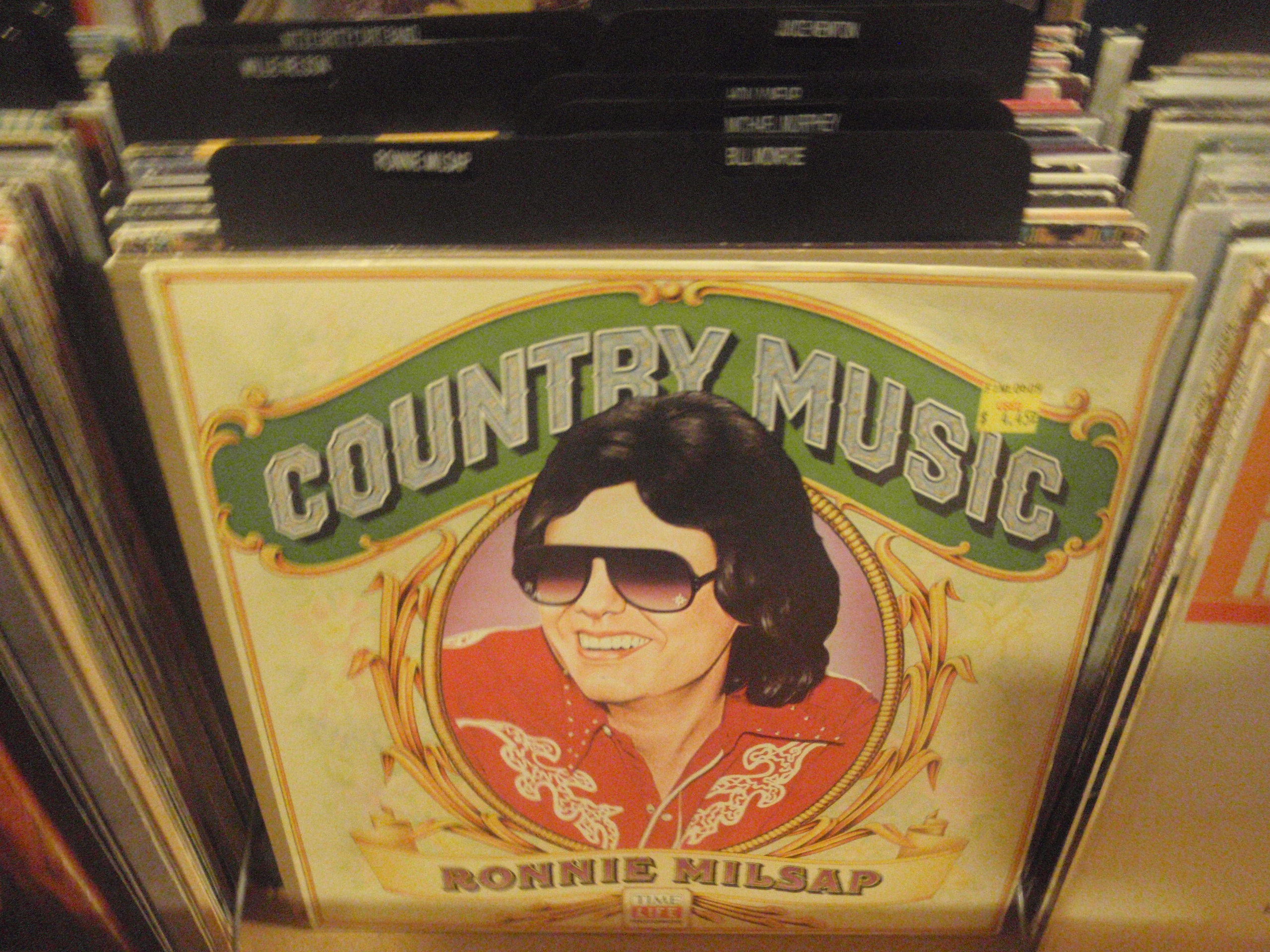The image depicts a vintage-style record store display with a grainy, orangey light ambiance. The central focus is on a prominently featured album titled "Country Music" with a green background and a gold decorative border. The album cover showcases a cartoon-like image of a smiling man with shoulder-length dark brown curly hair, wearing black aviator sunglasses and a red cowboy shirt with white detailing. This man is Ronnie Milsap, as indicated on a scroll beneath his picture, alongside a Time Life logo. The album, priced approximately at $4.45 as per a visible yellow sticker, is part of an A to Z organized stack of records. Behind it, dividers label the artists, including blurred names like Bill Moore and Michael Warren. The display evokes a nostalgic, vintage feel with numerous other records stacked on either side.